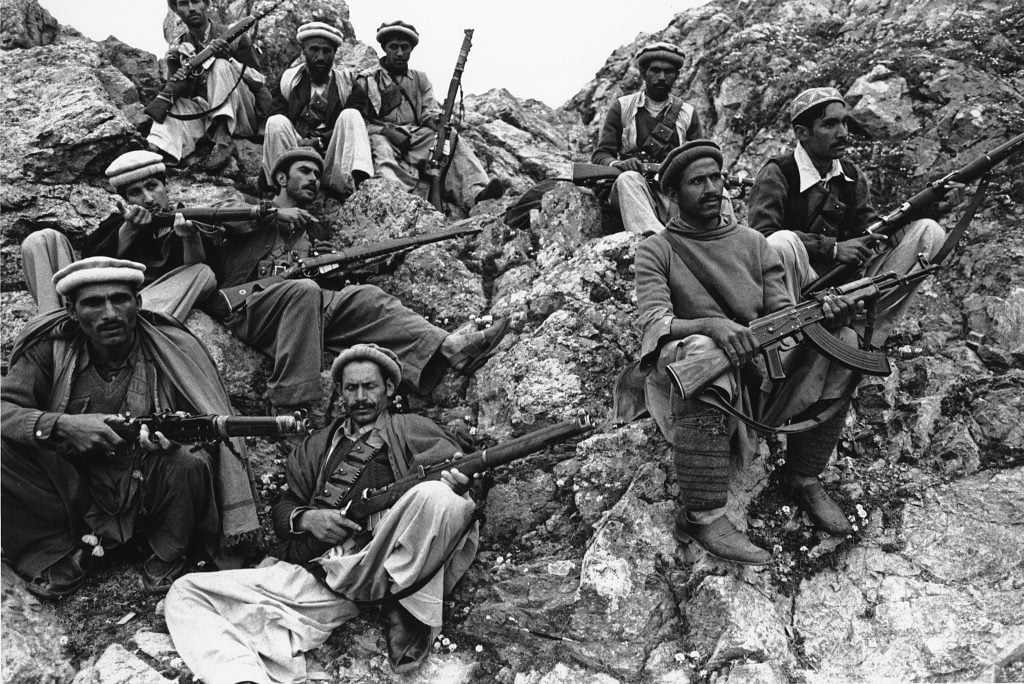This black and white outdoor image captures a group of weary, intense-looking men, possibly soldiers, nestled among jagged, craggy rocks. Each man, adorned with facial hair and wearing circular headgear, is equipped with a gun, predominantly machine guns and rifles, some pointed ahead while others rest at their sides. The scene, devoid of sunlight, presents a darker, more somber tone as they sit, kneel, and crouch on the rocky terrain, appearing fatigued and on high alert, scanning the distance as if anticipating someone's arrival. The rocky landscape occupies most of the frame, with a glimpse of a washed-out sky in the upper part of the image. The men, all dressed in long sleeves, trousers, and boots, exude a sense of readiness and vigilance amidst the harsh, rugged backdrop.